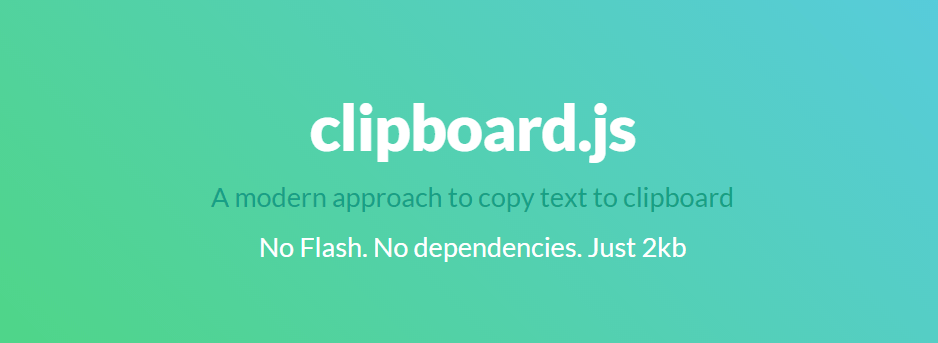The image features a screen displaying promotional content for Clipboard.js, an efficient tool designed for copying text to the clipboard. The central message, prominently written in thick white print font, reads "Clipboard.js". Below this, in a slightly darker greenish-gray hue, the text touts the tool's modern approach with the phrase, "a modern approach to copy text to clipboard." Further down, in white text of comparative or slightly larger size, reads the benefit statement: "No Flash. No dependencies. Just 2KB," with "Flash" uniquely capitalized.

The background of the rectangle transitions smoothly in a gradient from green on the left to a teal blue on the right, providing an aesthetically pleasing backdrop. The overall design is streamlined and modern, reflecting the efficiency and simplicity of Clipboard.js. Noteworthy are the lowercase 'k' and 'b' in "2KB," indicating the file size, giving an impression of compactness and functionality.